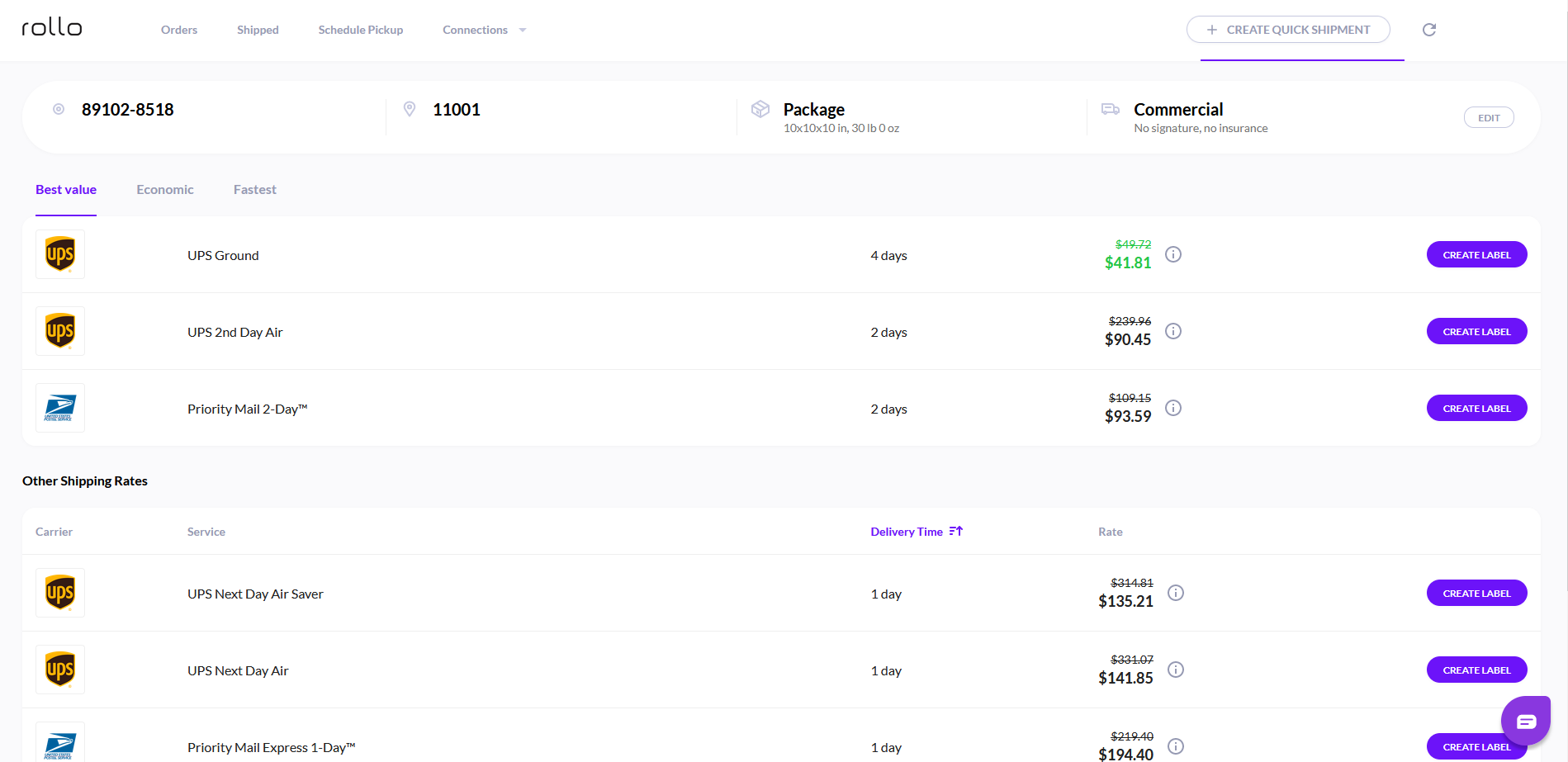This screenshot captures the user interface of a shipping platform. In the top left corner, "Rollo" is displayed prominently, with tabs to the right labeled "Orders," "Ship," "Schedule," "Pick Up," and a drop-down menu titled "Connections." On the left side, there is a button labeled "Create Quick Shipment" followed by a refresh button. Beneath these buttons is a purple line.

The lower part of the interface shows detailed shipping information. Starting from the left, it lists a number: "891028518", a location code: "11001", and the package dimensions: "10 x 10 x 10 inches". The package weight is listed as "0 ounce," and it is specified as non-commercial, with no signature required and no insurance.

In the bottom left, a table compares shipping options under tabs such as "Best Value," "Economic," and "Fastest." The "Best Value" tab is selected and highlighted in purple. This section details various shipping options:

- **UPS Ground:** Delivery in 4 days for $41.81 (highlighted in green as a cheaper option), with a "Create Label" button.
- **UPS Second Day Air:** Delivery in 2 days for $90.45, discounted from $239.96, also featuring a "Create Label" button.
- **Priority Mail 2-Day:** Delivery in 2 days for $93.59, reduced from $109.15.

Below, additional shipping rates are displayed:

- **UPS Next Day Air Saver:** Delivery in 1 day for $135.21, discounted from $114.81.
- **UPS Next Day Air:** Delivery in 1 day for $141.85, reduced from $301.07.
- **Priority Mail Express 1-Day:** Delivery in 1 day for $194.40, discounted from $290.40.

Each shipping option includes a "Create Label" button, characterized by the purple color.